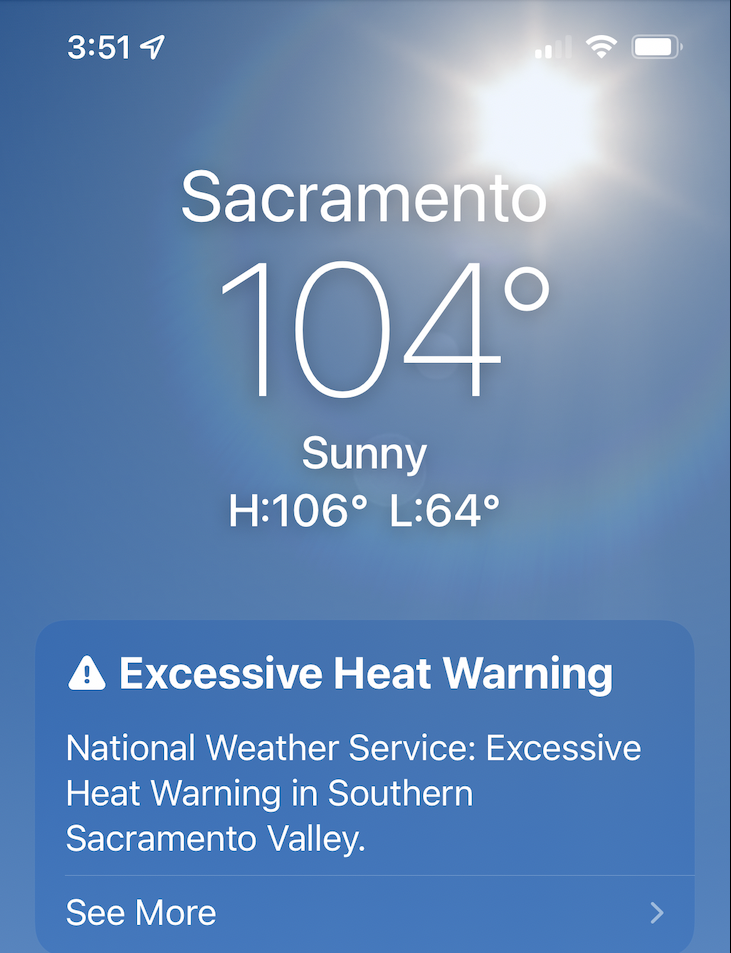The image depicts a smartphone screen displaying various weather-related information. In the upper left corner, the time is shown as 3:51 PM. Adjacent to this, on the upper right side, there are icons indicating full Wi-Fi signal strength and battery level.

Prominently in the center, the screen displays the location "Sacramento" in a bold font size of 104, with the temperature reading 104 degrees Fahrenheit. Below this, it gives additional temperature details, noting a high of 106 degrees and a low of 64 degrees.

Underneath this information, there is a blue rectangular box featuring a white triangle with an exclamation point inside. This graphic is accompanied by the text in bright white indicating "Excessive Heat Warning," issued by the National Weather Service for the southern Sacramento Valley. A thin line beneath this text leads to an option labeled "See More," marked by a right-pointing arrow, both in a lighter shade of blue.

The background of the screen showcases a sunny sky, with a vividly bright sun located in the upper right corner. The sun emits six radiant rays and has a halo effect. The predominant colors used in the image are various shades of blue, white, and some yellow-orange hues for the sun rays.